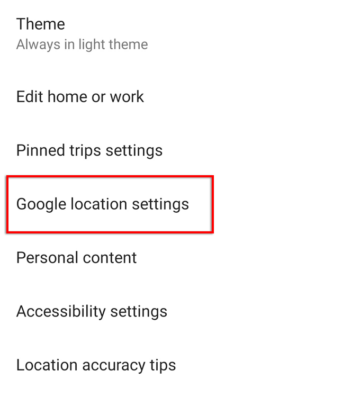The screenshot displays a settings menu against a white background, which seems to follow a consistent white theme. The options available in the menu include "Edit home or work," "Pintrip settings," "Google location settings"—this particular option is emphasized with a red rectangle around it—"Personal content," "Accessibility settings," and "Location accuracy tips." The image highlights the "Google location settings" element, suggesting it is the focus of attention or something requiring user action.